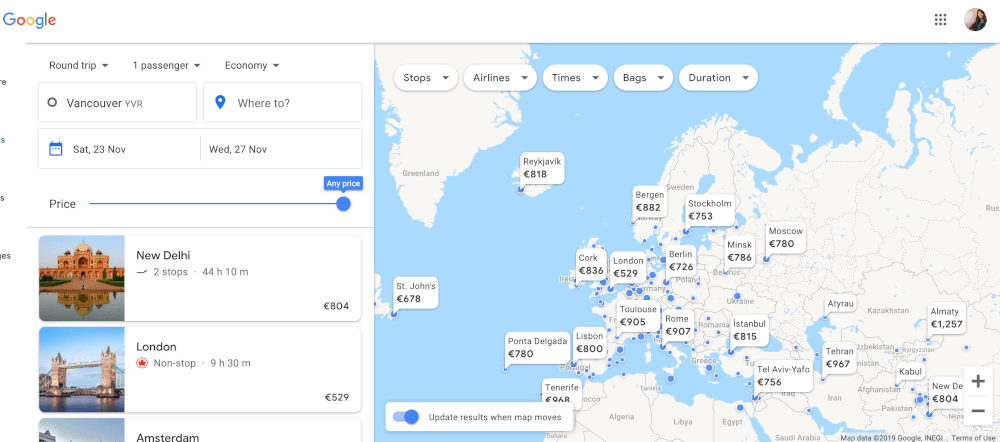Screenshot of a Google Flights search page displaying round-trip flight options, pricing, and a map. The search parameters are set for one passenger in economy class, flying round trip from Vancouver to destinations unknown, with travel dates from Saturday, November 23 to Wednesday, November 27. Below the search form, two highlighted flight options are shown: New Delhi with two stops (illustrated with a photo of an old-style building by a lake) and London with a non-stop flight (illustrated with a photo of a large bridge).

To the right of the flight options is a detailed map encompassing much of Europe, parts of North Africa, and segments of Eastern Europe and Greenland. Key locations and their round-trip prices in euros are marked: St. John's (€678), Lisbon (€800), Rome (€907), and Istanbul (€815). Countries labeled on the map include Sweden, Belarus, Ukraine, Germany, Algeria, Libya, and Egypt. An option to update results as the map moves is activated at the bottom left corner of the map.